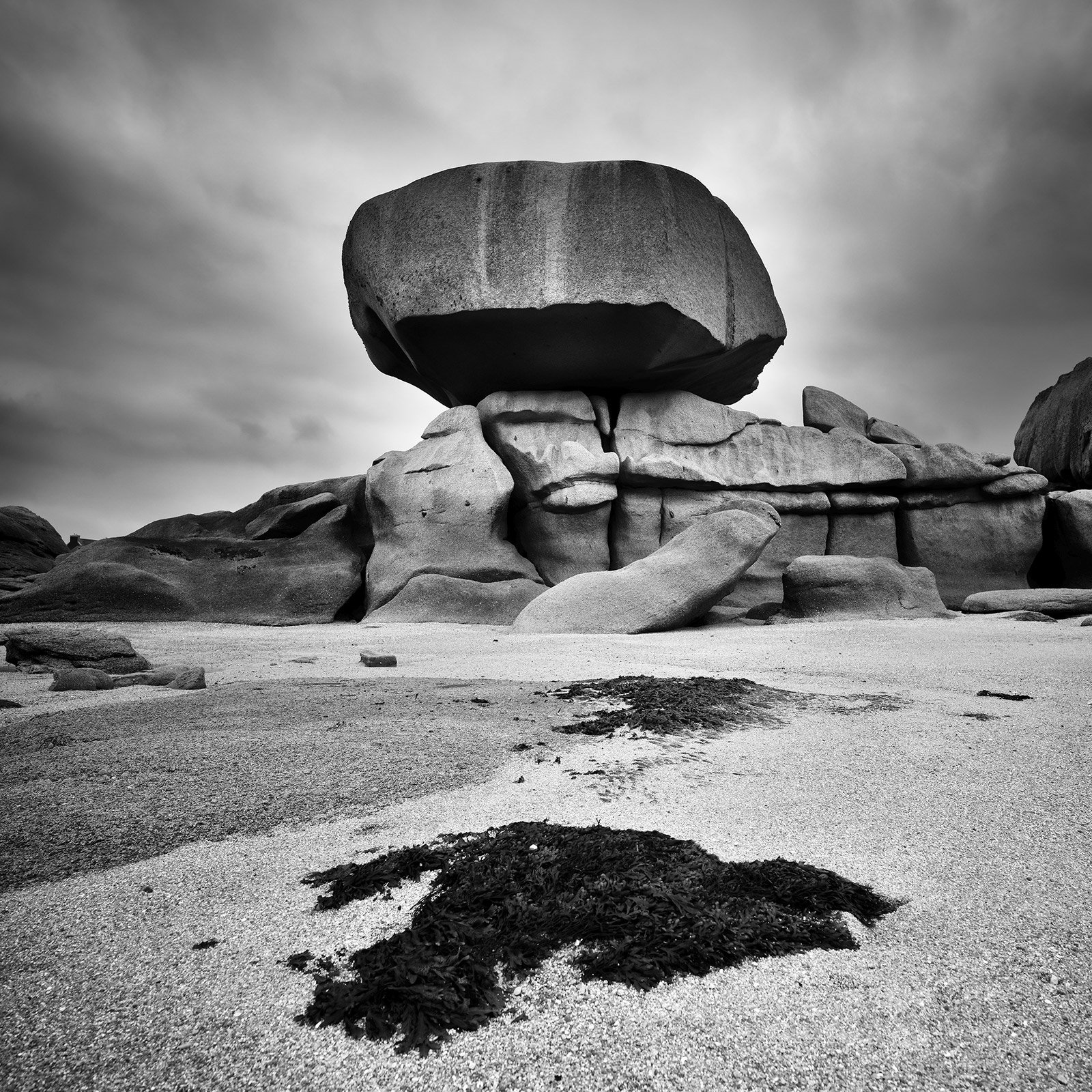A monochromatic photograph captures an outdoor scene featuring a massive boulder precariously balanced atop a cluster of large rocks. The ground in the foreground is sparsely covered with small piles of dark mulch, which is also scattered towards the middle of the image. The rest of the terrain is a mix of sand and dirt, creating a rough and textured surface. The sky overhead is filled with clouds, adding a moody atmosphere to the black-and-white palette, emphasizing the stark contrast and dramatic nature of the landscape.